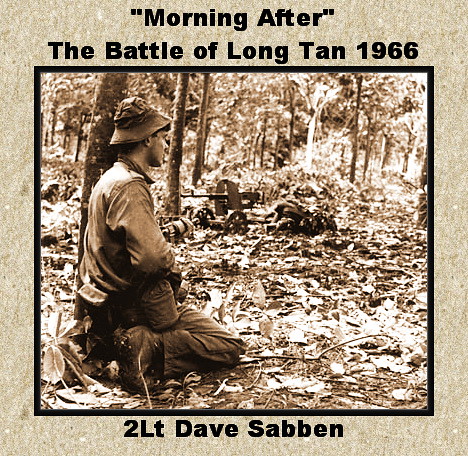This detailed sepia-toned photograph is framed by a dark black border and set against a tan background with an aged, textured appearance resembling browning paper. The central image captures Second Lieutenant Dave Saban, a soldier in the aftermath of the Battle of Long Tan in 1966, as specified by the black text captions at the top and bottom of the border. Saban, dressed in army fatigues and a bucket hat, is kneeling in a woodland area filled with dead leaves and twigs; his body is angled away from the camera while his face is shown in profile. The scene appears to depict a moment of calm amid the chaos, with indistinct military equipment, possibly artillery and helmets, scattered in the background.